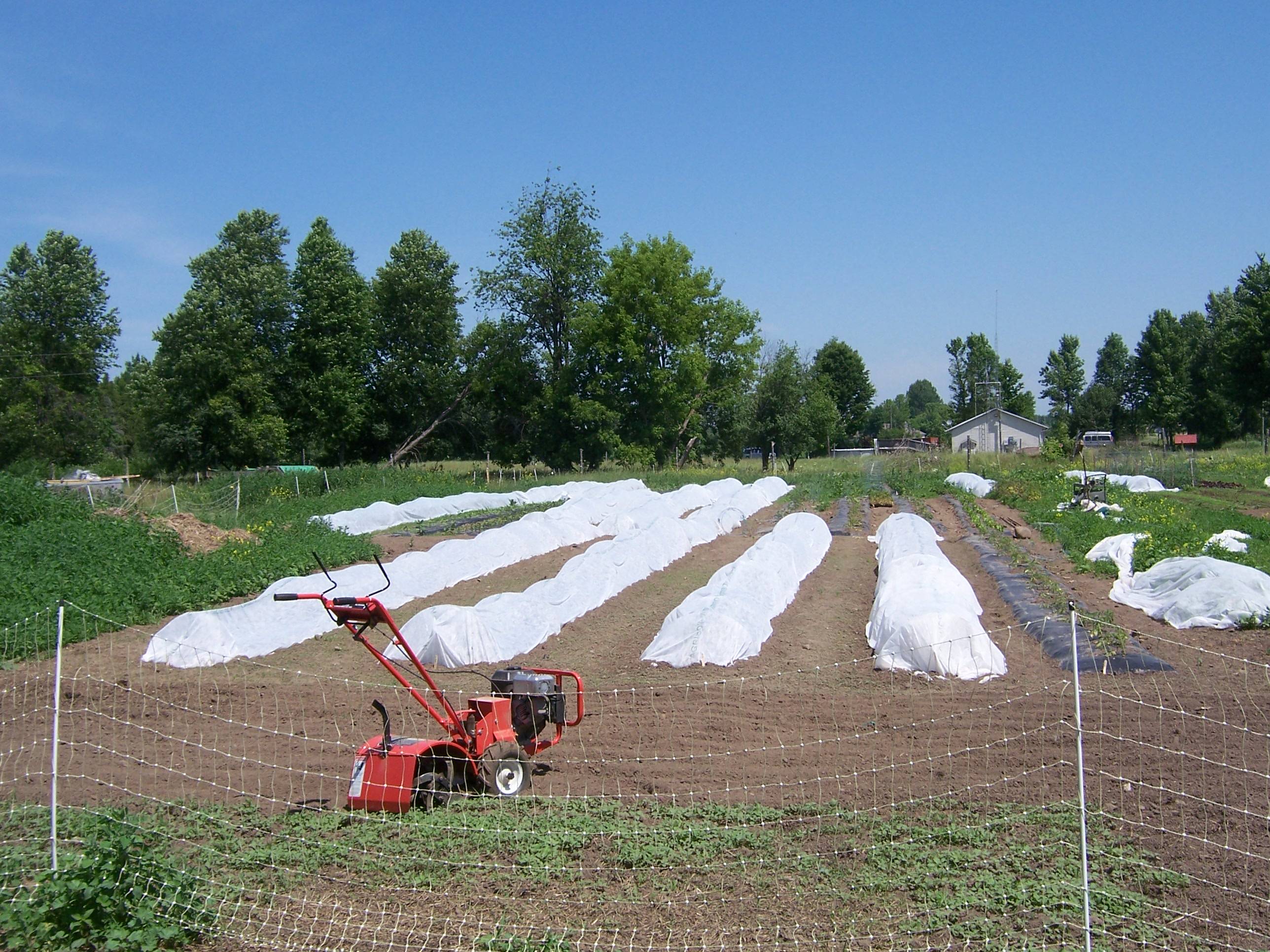This is a detailed color photograph of a farm field taken outdoors during the daytime, showcasing both cultivated and uncultivated areas bathed in natural light. In the background, a series of trees forms a natural border, accompanied by a house with a van parked to its right, all beneath a clear, blue sky graced with a few clouds. In the midground, rows of raised garden beds stretch into the distance, some covered with white tarps while others remain uncovered, revealing plants growing among them. The entire field is predominantly bare dirt, with the exception of a grassy region on the right and lush, overgrown vegetation on the left-hand side.

In the foreground, a wire fence with white posts runs horizontally across the scene, partially enclosing the area. On the bottom left, a red rototiller equipped with large black tires and bright orange handles sits idle, not in operation. Another similar piece of machinery can be spotted in the grassy area to the right. The overall composition highlights the blend of human cultivation and natural growth, framed by the orderly rows of garden beds and the untamed grass along the periphery.